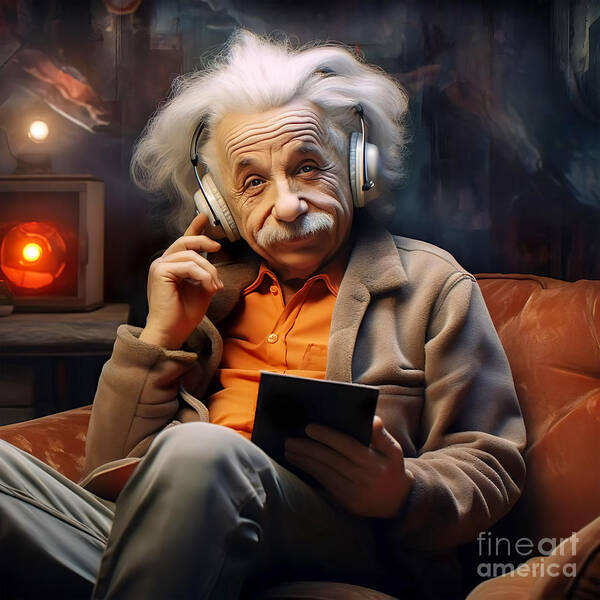This meticulously detailed image features a CGI representation of Albert Einstein comfortably seated on a cushioned, velvety orange lounge chair. His iconic poofy white hair and bushy mustache are perfectly captured, enhancing his recognizable demeanor. Einstein is depicted wearing modern white headphones with teal ear pads, giving a nod to contemporary times. He is dressed in an orange button-down shirt with a collar, gray pants, and a fuzzy, light brown jacket, exuding a laid-back yet intellectual vibe. His right elbow is bent, with his pointer finger thoughtfully touching the right side of his headphones. Einstein's body is angled towards the lower portion of the image, while his face is turned forward, showcasing his signature smile as he engages with the camera. The background subtly includes a table with some lights, adding to the modern ambiance. The image's high resolution and clear lighting suggest a sophisticated AI-generated creation. In the lower right corner, the watermark "Fine Art America" is visible, and the left corner has a mysterious blend of orange and white light beaming out, adding to the unique visual appeal of this striking artwork.